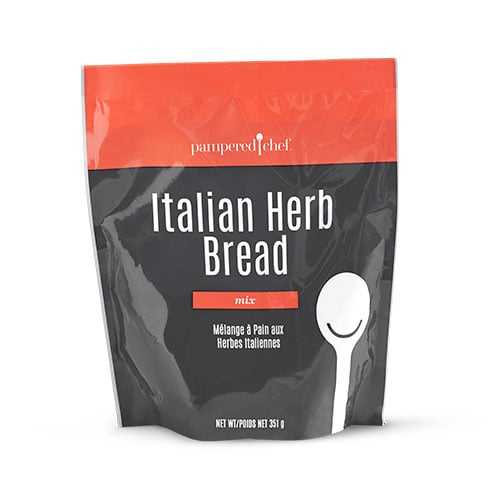The photograph showcases a glossy, rectangular plastic bag set against a white background, reminiscent of a product image you'd find on Amazon. The upper portion of the bag features a prominent red horizontal stripe, which includes the white text "Pampered Chef" and a white spoon icon between the words. Below this red stripe, the majority of the bag is a dark gray or black. Centered on this dark background, large white text reads "Italian Herb Bread." Underneath this, a horizontal red rectangle contains the word "Mix" in white text. Below this red bar, smaller white text says "Melange à Pain aux Herbes Italiens." Towards the bottom of the bag, also in white text, it indicates a net weight of "351 grams." On the right side of the packaging is an illustrated white spoon with a curved top and thin handle, adding a touch of detail to the design. The overall presentation of the bag is shiny and visually distinctive, with the top quarter in red and the lower three-quarters in dark gray or black.